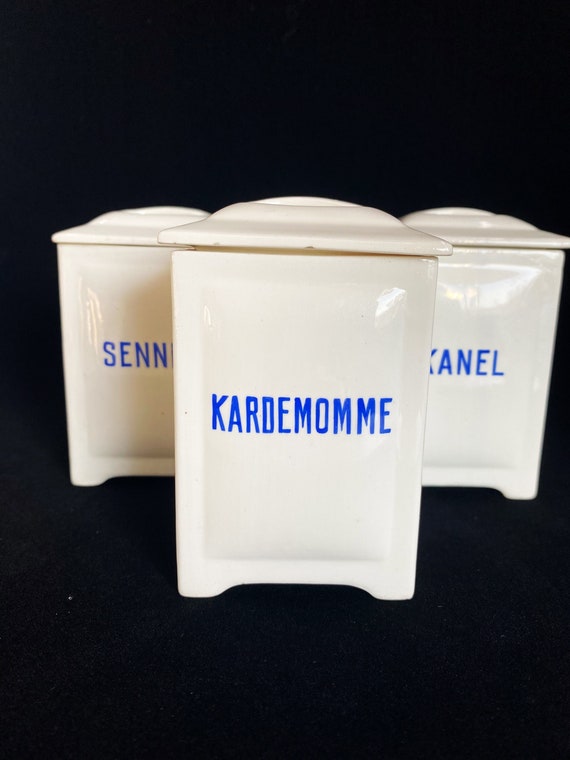This is a horizontally aligned rectangular image featuring three white spice containers against a solid black background. The containers, either glass or ceramic, are vertical and rectangular with tops resembling small lids that can be removed. They stand on short, stubby legs. The white surface of each container has blue, all-caps text painted on them. The container in the foreground prominently displays "KARDEMOM" spelled "K-A-R-D-E-M-O-M-M-E." Behind this, partially obscured, the left container reads "SENN," and the right one reads "KANEL," though the beginning of each word is blocked by the front container. The detailed image, reminiscent of porcelain or clay craftsmanship, shows the containers resting on what looks like black cloth.